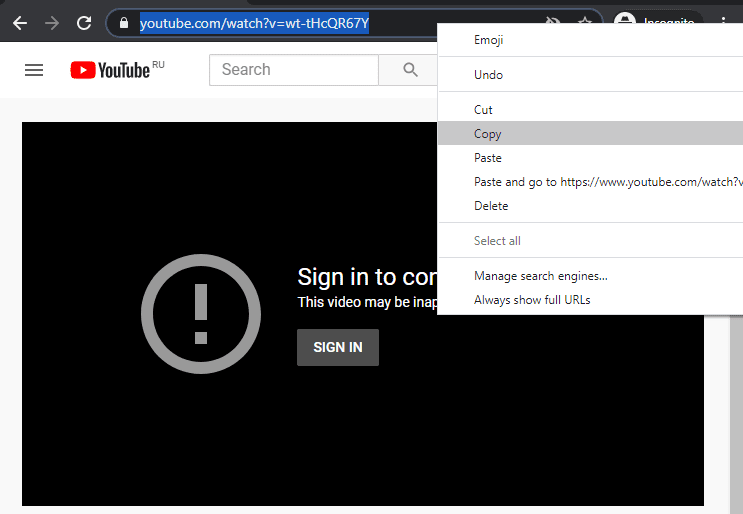**Detailed Caption:**

The image is a screenshot of a YouTube video page displayed within the Google Chrome web browser, operated in incognito mode. The URL in the address bar reads youtube.com/watch?v=WT-THcQR67Y, and this link is highlighted in blue. The user has right-clicked on the URL, opening the context menu with the intention to copy the video link. In the background, YouTube prompts the user to sign in, indicating that the video content may be inappropriate for certain audiences. This screenshot might be illustrating a method to bypass the sign-in requirement, potentially for those who prefer not to share personal information online to maintain privacy.